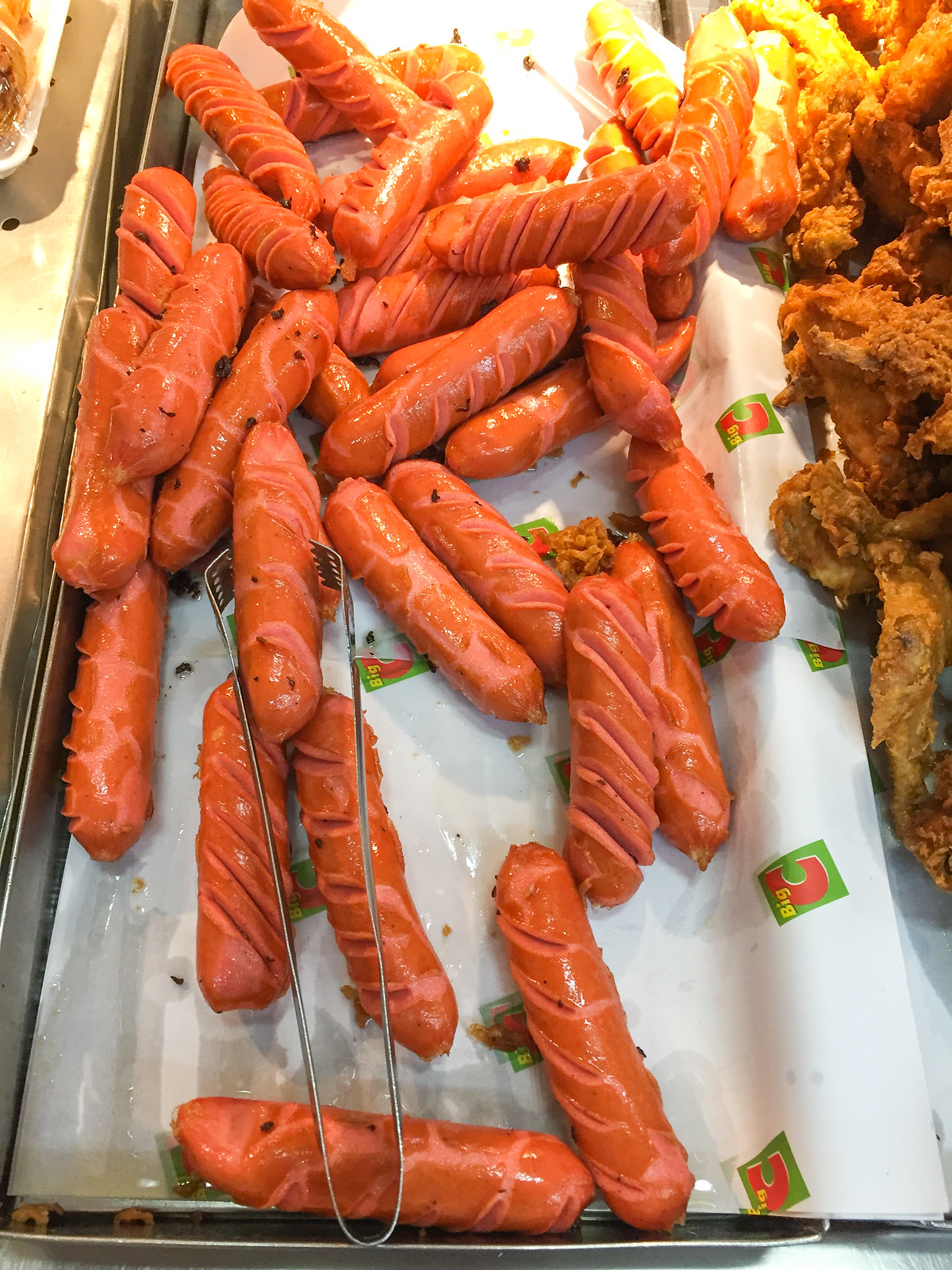The image captures a buffet setup featuring a variety of foods displayed in a large metal tray lined with white parchment paper, branded with a "Big C" logo in yellow and red text on a green square background. Central to the image are numerous small hot dogs or sausages laying closely together, distinguished by orange-brown cooked casings and diagonal slits running along their lengths. A pair of silver steel tongs with tines is positioned gripping one of the hot dogs. To the right, there are pieces of golden brown, crispy fried chicken or similar breaded meat. Another level of silver display is visible in the top right, suggesting additional food items under what appears to be bright overhead lighting, enhancing the cafeteria-like or restaurant ambiance.